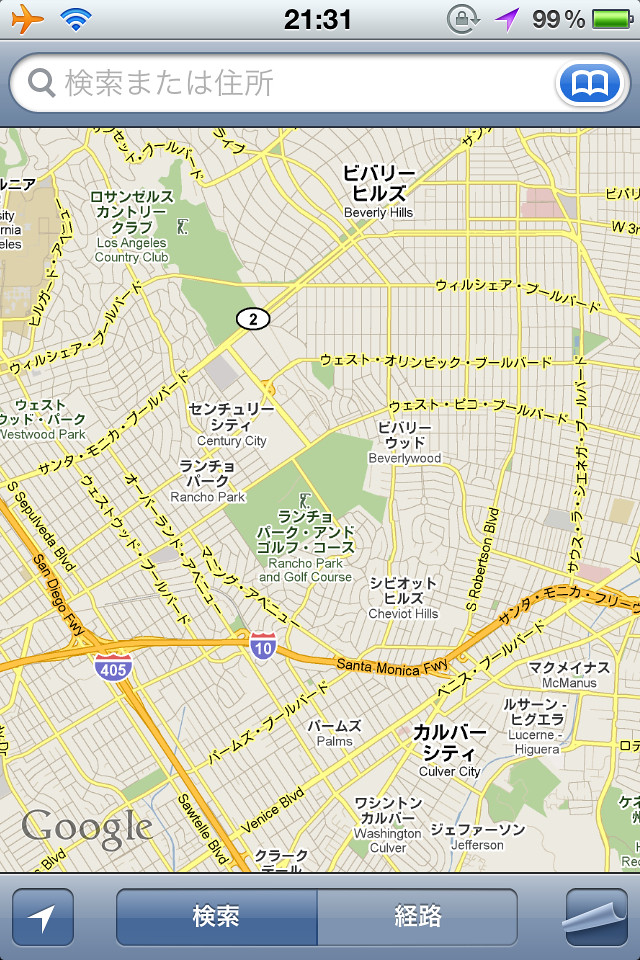This image is a detailed screenshot of a map interface. 

At the top of the image, there is a vertical gray column, followed by a long rectangular row. In the top left corner, an orange airplane icon is visible. Next to it is a symbol comprising three blue lines and a triangle. Prominently displayed in the center of the top row is the number "2131." Additional symbols include a small icon featuring a circle with an arrow and a lock, a purple arrow with a "99%" indicator, and a green battery symbol.

Beneath this top row is another gray box with a central white circle that spans the width of the box. Within this circle, there is a gray magnifying glass and some Chinese characters. An adjacent oval features a blue background with a white book icon.

The main portion of the image displays a map, predominantly yellow, with various hues and colors to differentiate features: yellow for roads, green for parks, and darker yellow for side roads and interstates. The map is densely packed with a network of roads, indicative of a city layout.

At the bottom of the image, there is another gray line containing multiple square icons. On either end of this line are squares, with two additional squares positioned in the center. The first square includes an arrow, while the two central squares feature Chinese writing. The final square resembles a piece of paper being pulled up.

Overall, the map interface is highly detailed, with numerous navigational elements and symbols designed to aid in urban navigation.